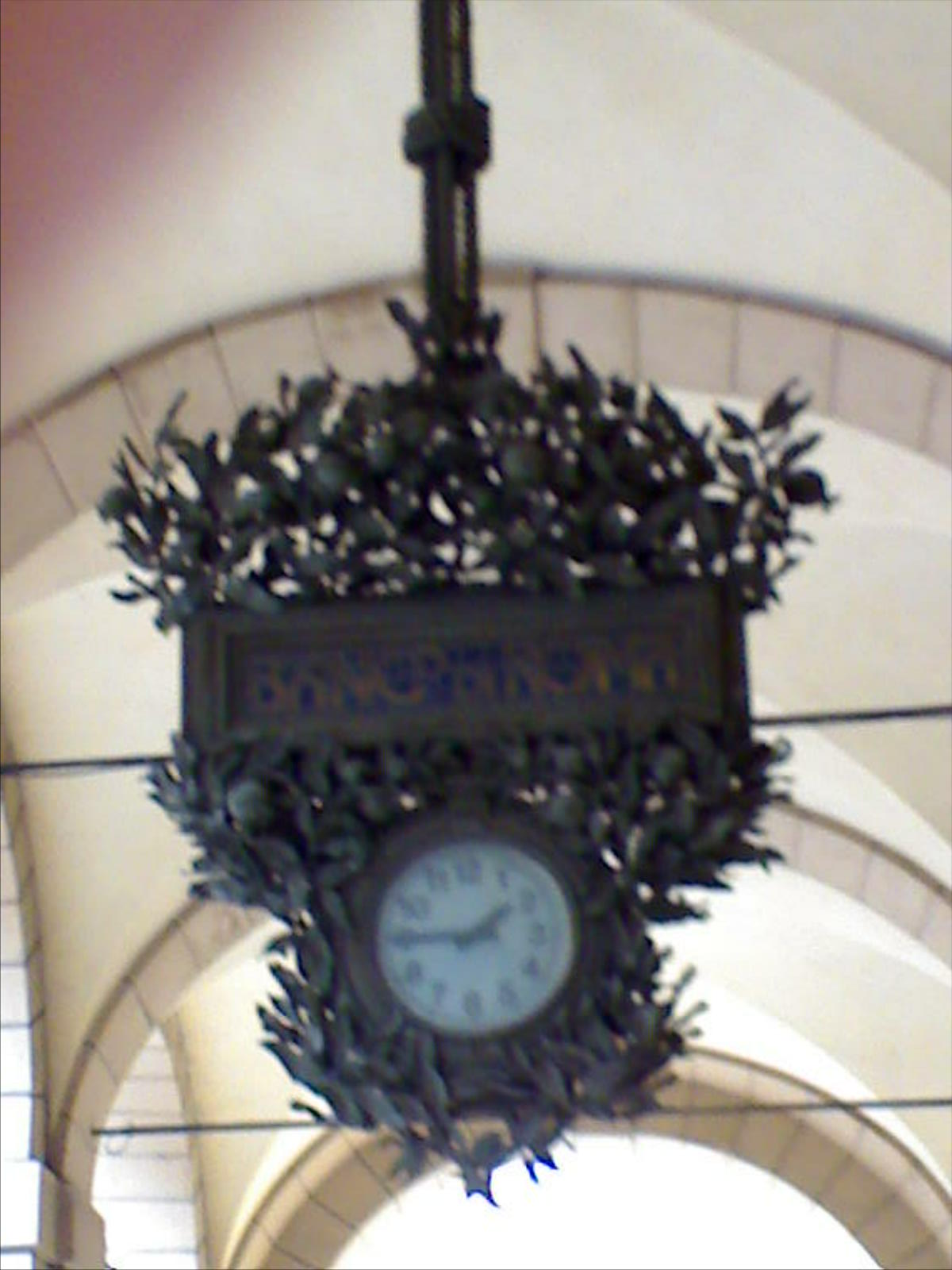A close-up photograph captures a unique clock hanging from the ceiling of a public building. The clock, adorned with a green, leafy design, exudes an elegant yet organic aesthetic. Suspended above are three tent-like structures, adding architectural intrigue to the space. The clock itself is somewhat blurred, making the details challenging to discern. It features a white face with numerals encircling it, and above the clock, there is a blue panel with gold lettering that appears to spell "BANOPANOMA," although the text is difficult to read clearly due to the blur. The overall image offers a glimpse into a richly detailed and thoughtfully designed public space.